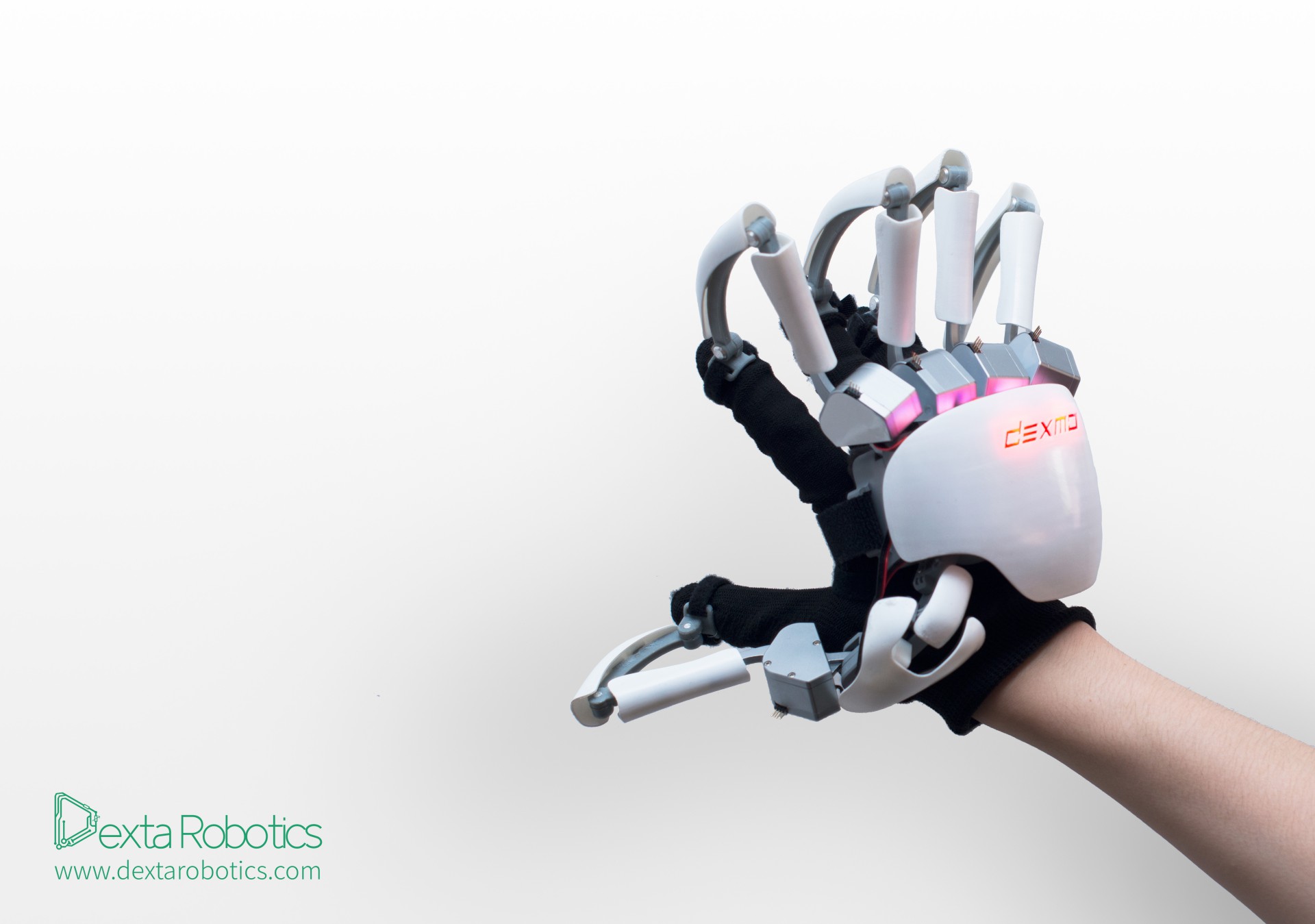The photograph showcases a human forearm emerging from the lower right corner, angled upwards toward the upper left. The forearm is adorned with a black glove featuring a white robotic exoskeleton that encompasses the palm and fingers. This advanced prosthetic device, labeled "Dexmo" on the back of the palm, integrates seamlessly with the hand, resembling a skeletal structure with metallic rods and joints visible. The knuckles are accentuated by pink lights, adding a cybernetic flair to the design. The exoskeleton's fingers are linked to individual silver connectors, while a thumb component extends horizontally, also featuring white casing and metal joints. The background is a clean white, emphasizing the futuristic aesthetic of the prosthesis. In the bottom left corner of the image, "Dexter Robotics" and the website "www.dexterrobotics.com" are prominently displayed in green text.